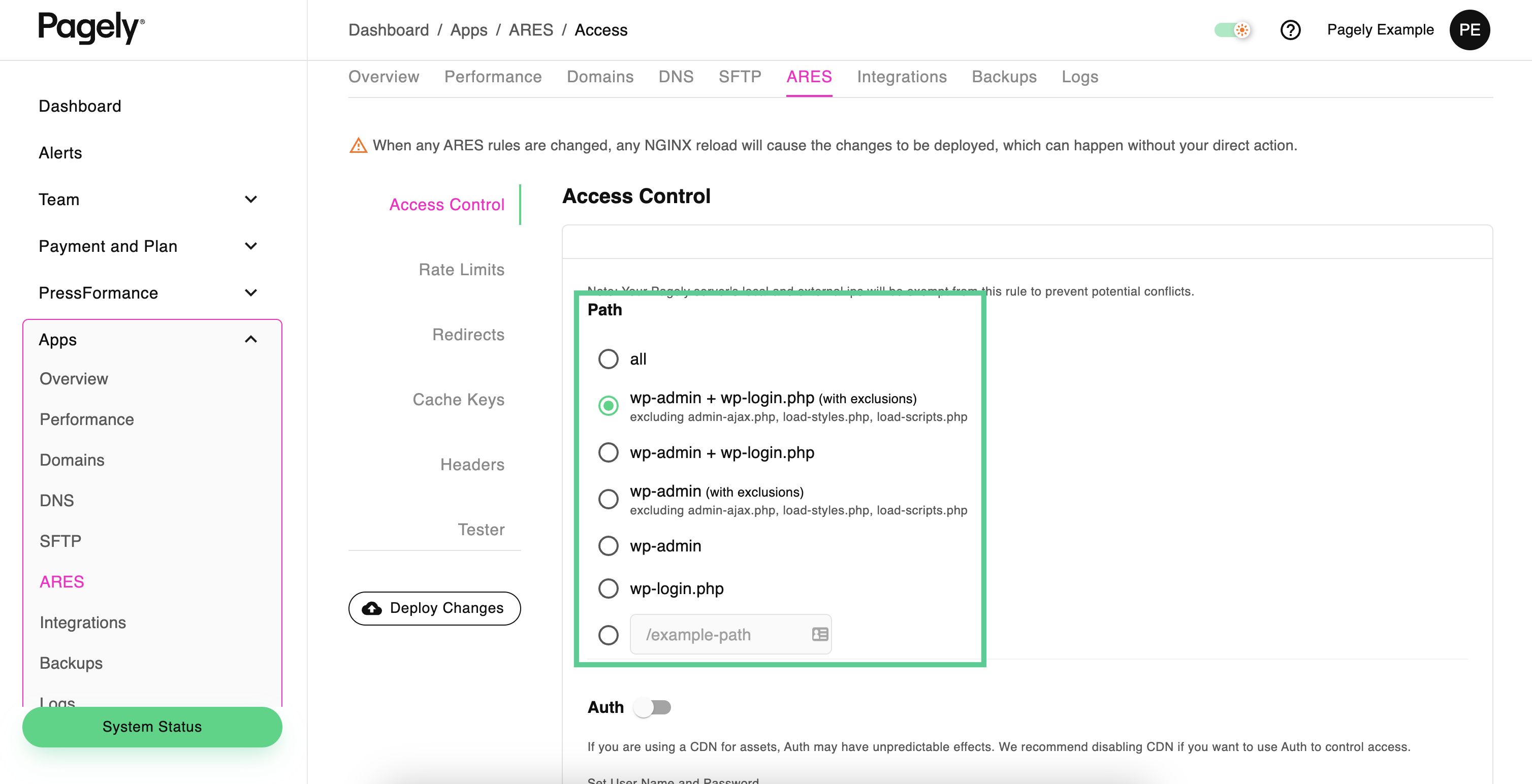**Caption:**

This screenshot displays a detailed view of the Pagely web interface, specifically highlighting the "Access Control" section. 

- At the top left corner, the Pagely logo is prominently displayed in black letters ("P-A-G-E-L-Y").
- Directly underneath, a vertical menu lists various sections including: Dashboard, Alerts, Team, Payment and Plan, Pressformance, Apps, Overview, Performance, Domains, DNS, SFTP, Ares, Integrations, Backups, Logs, and System Status. 
- To the right, a horizontal menu mirrors several of these options: Dashboard, Apps, Ares, Access, Overview, Performance, Domains, DNS, and SFTP. The "Ares" section is selected, revealing options specific to it.
- Upon any changes to Ares rules, an NGINX reload ensures these changes are deployed even without direct user action.
- A secondary vertical menu appears with options: Access Control (selected), Rate Limits, Redirects, Cache Keys, Headers, Tester, and Deploy Changes.

The main content area focuses on the "Access Control" settings:

- An outlined green box lists path configurations, with options such as "All," "WP-Admin plus WP-Login.php (with exclusions of admin-ajax.php, load-styles.php, and load-scripts.php)," "WP-Admin," "WP-Login.php," and a custom path "example-path."
- The selected radio button currently highlights "WP-Admin plus WP-Login.php with exclusions."
- The interface notes that enabling authentication ("Auth") might have unpredictable effects if using a CDN for assets, recommending disabling CDN to use Auth effectively. 

This comprehensive view of the Pagely interface offers insights into the configuration and control options available for advanced website management.